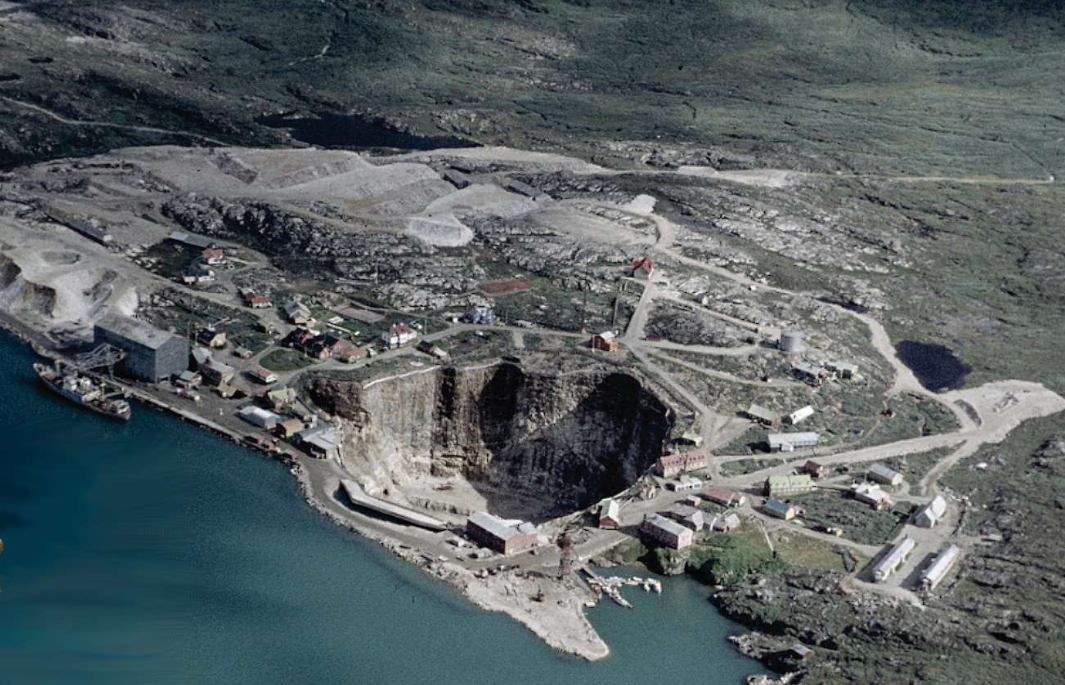This aerial shot captures a massive quarry adjacent to a body of water in the bottom left-hand corner. The calm blue water features a long ship moored at a pier, next to a large warehouse. The shoreline transitions into a vast expanse of land dominated by the deep and expansive quarry, characterized by sheer drop-offs and rugged cliff sides. Small buildings of varying sizes, predominantly white with red roofs, are scattered across the site, connected by dirt-brown roads. Gravel and other materials are piled up around the area, indicative of ongoing excavation. Vegetation surrounds parts of the quarry, contrasting with the barren, gravel-laden interior. Despite the clear presence of human activity, the specific location remains unidentified.